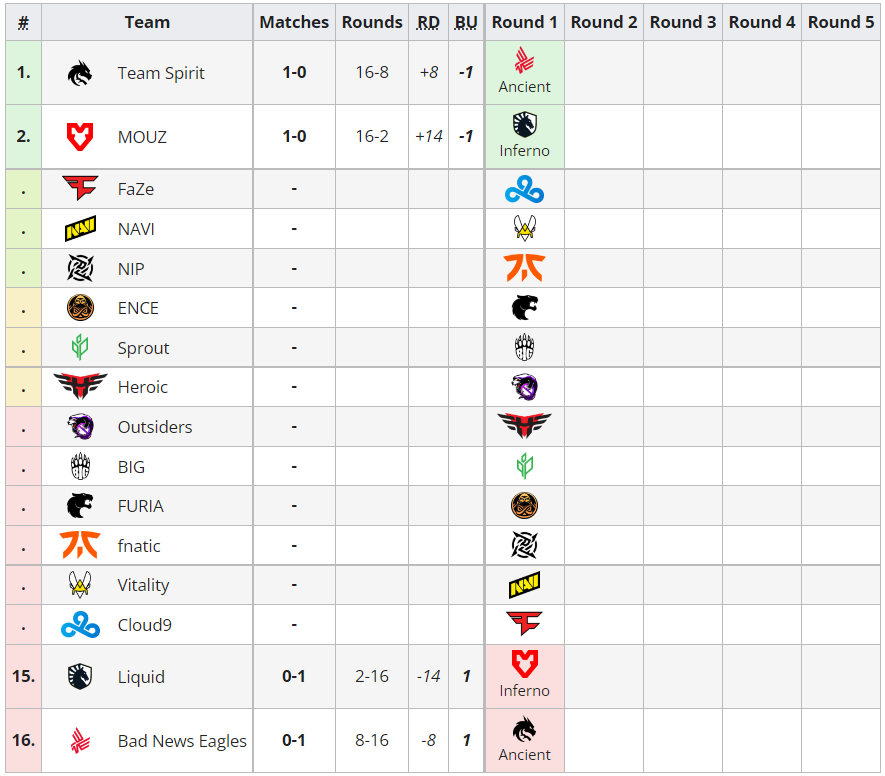The image depicts a detailed table of a sports tournament, possibly for a match with multiple rounds. Across the top row of the table, each column is titled respectively: Number, Team, Matches, Rounds, RD, BU, Round 1, Round 2, Round 3, Round 4, and Round 5. 

On the left-hand side, starting from the first column, the numbers sequentially list the teams. Each row alternates between light gray and white for better readability. Here's a detailed look at the content:

- **Row 1:** 
  - Number: 1
  - Team: Team Spirit
  - Matches: 1-0
  - Rounds: 16-8
  - RD: +8
  - BU: -1
  - Round 1: Highlighted in green, labeled "Ancient" with an accompanying symbol representing another team.

- **Row 2:**
  - Number: 2
  - Team: Mals
  - Matches: 1-0
  - Rounds: 16-2
  - RD: +14
  - BU: -1
  - Round 1: Highlighted in green, labeled "Inferno."

Following these rows, other listed teams include: 
- **Row 3:** Phase
- **Row 4:** Navi
- **Row 5:** Nip
- **Row 6:** Entz
- **Row 7:** Sprout
- **Row 8:** Heroic
- **Row 9:** Outsiders
- **Row 10:** Big
- **Row 11:** Furia
- **Row 12:** Fnatic
- **Row 13:** Vitality
- **Row 14:** Cloud9
- **Row 15:** Liquid
- **Row 16:** Bad News Eagles

The format of the table clearly shows the performance metrics of each team across different rounds, providing a comprehensive overview of the tournament’s progress.